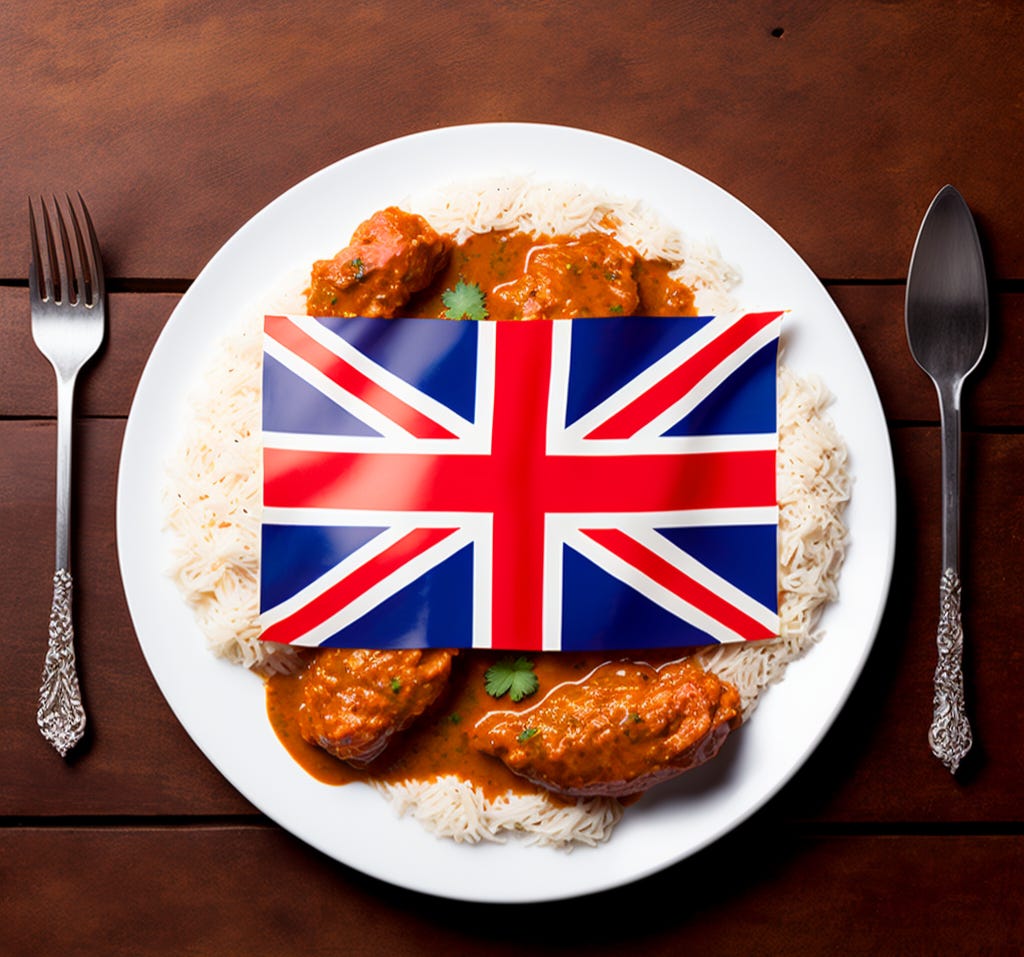The image appears to be a hyper-realistic digital illustration of a dinner plate featuring a serving of butter chicken with white rice. The scene is set on a surface that resembles brown leather. The white plate is centered in the image, showcasing a bed of thin long-grain white rice topped with several pieces of chicken enveloped in an orange-red sauce. Garnishing the dish are petite cilantro leaves, adding a touch of green contrast. Intriguingly, a small flag designed to resemble the Union Jack is placed on top of the food, though it is not an accurate representation.

On either side of the plate, there are utensils—a metal fork on the left and a spoon-like implement on the right. The fork has an unusual number of tines, possibly five or six, and they are inconsistently shaped. The spoon seems disproportionately narrow, almost like a short knife, making its true function ambiguous. Both implements, along with the plate, are arranged on what looks like a wooden or leather-textured table, adding a rustic touch to the overall composition.